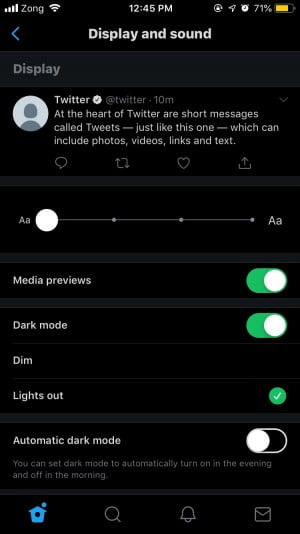The image displays a smartphone screen with a detailed view of the Twitter application's settings. At the very top, the status bar indicates the network provider "Zong" alongside several symbols: Wi-Fi, time, clock, and battery percentage.

Below the status bar, the screen header features a blue back arrow next to the title "Display and Sound". Under the "Display" category, the subheading "Twitter" is prominently shown, accompanied by the label "@Twitter" and a time entry of "10 minutes". 

A white text block explains: "At the heart of Twitter are short messages called tweets, just like this one, which can include photos, videos, links, and text." This description is followed by an array of familiar interaction icons: reply, retweet, a heart for liking, and a share button.

Further down, a font size adjustment scale is visible, starting with a smaller "AA" on the left, a white adjustable circle, and a larger "AA" on the right, allowing users to increase or decrease text size. 

Several toggles and checkboxes are listed under additional settings:
- "Media previews" has a green indicator showing it is turned on.
- "Dark mode" is also enabled with a green indicator.
- Options for "Dim" and "Lights out" both have green checkmarks.
- "Automatic dark mode" is currently off.

At the bottom, an informational note states: "You can set dark mode to automatically turn on in the evening and turn off in the morning."

The bottom navigation bar includes:
- A blue home icon.
- A white magnifying glass for search.
- A white notification bell.
- A white envelope icon for direct messages.